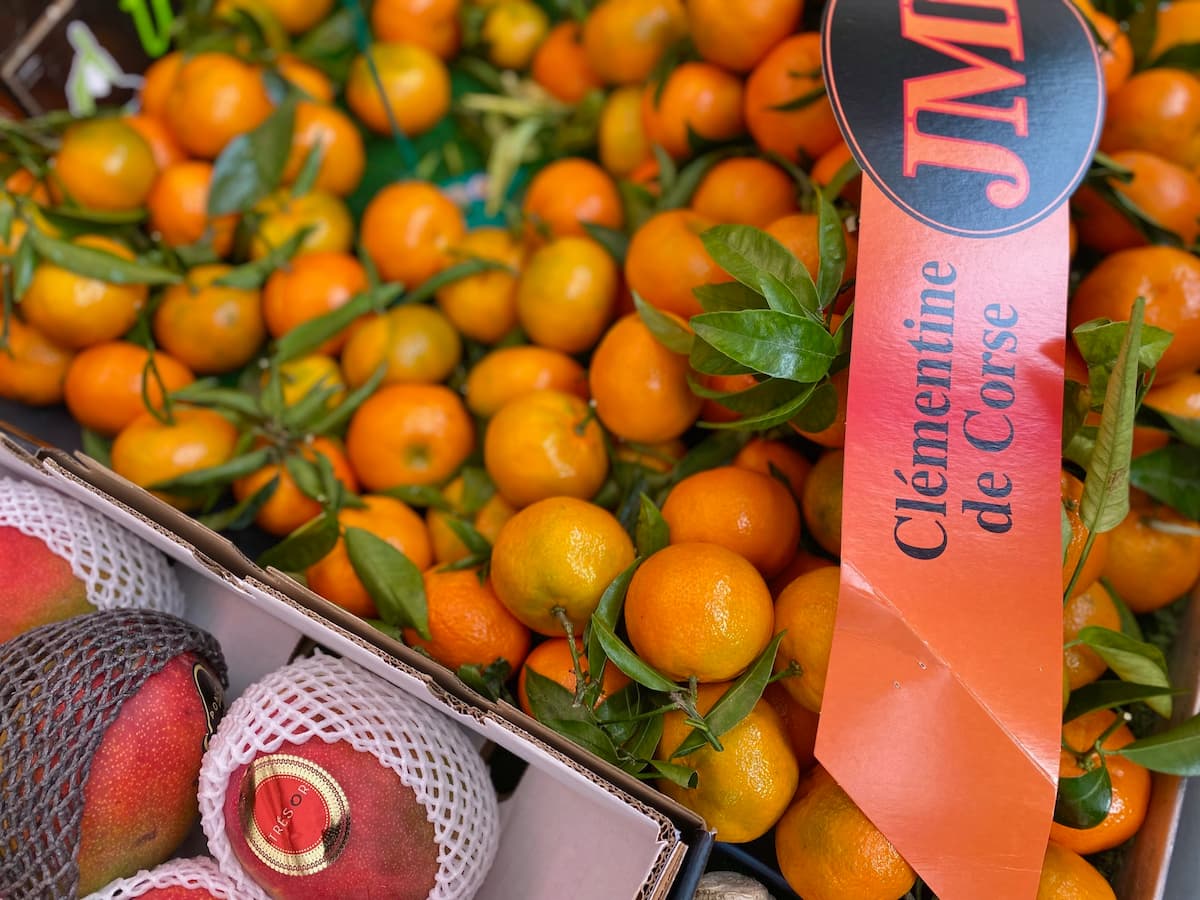In this detailed color photograph, we see a close-up view looking down into a vibrant fruit stand. Dominating the foreground is a pile of small clementine oranges, some of which still have their green stems and leaves attached. The orange skin of the clementines contrasts beautifully with the slight blur of others in the background, drawing our focus. At the top of this pile, a piece of orange paper bears the label "Clementine de Corse," with a black circle containing the letters "J-M." In the lower left corner of the image, part of a logo is visible. Nearby, in a cardboard box on the bottom right, are ripe mangoes, distinguished by their reddish-pink hue and each protectively wrapped in a soft, white, netted styrofoam bag. This composition emphasizes the freshness and careful presentation of the fruits, showcasing both clementines and mangoes in a visually appealing manner.